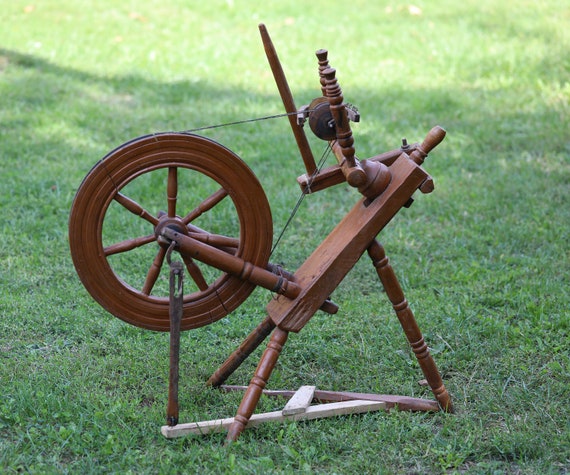This is a detailed photograph of a wooden machine set outdoors on a patch of green, trimmed grass. The machine, primarily composed of wood in various brown shades, consists of a central wheel or circular component that resembles a wheel spoke. Attached to this wheel are several strings or ropes, suggesting that it may function as a type of spinning machine for thread. The structure is supported by a combination of three to four wooden legs, with a base or board connecting the legs to ensure stability. Some descriptions mention a handle at the top, while others describe cylindrical wooden pieces and a second smaller circular element at the back, connected by poles. The overall scene is well-lit, indicating a sunny day.